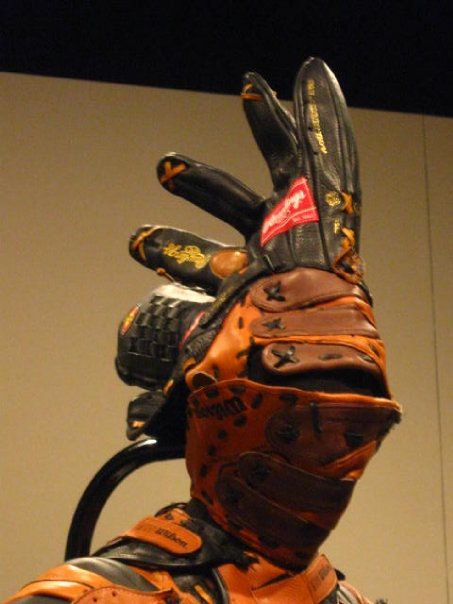The image features a fascinating sculpture resembling a knight's armor, meticulously crafted from various baseball gloves. The head of the figure appears to be fashioned from a dismantled baseball mitt, displaying a triangular headpiece with a visor slit, akin to a medieval knight's helmet. The helmet is composed of both black and orange gloves, prominently featuring brands like Rawlings and Wilson. A distinctive element is a black glove with yellow designs, creating a crest-like structure on top of the head, reminiscent of a rooster’s comb or an Indian headdress, with the fingers splayed out and flaring backward.

The upper portion of the statue, including the shoulders, is also constructed from baseball gloves reconfigured to imply a sturdy armor-like appearance. The gloves, primarily in shades of orange, light brown, black, and some accents of gold, are intricately stitched together, with visible brand logos such as Wilson in black writing and Rawlings in red and white.

Supporting the figure is a black bar that extends from the back of its neck and curves behind the head, giving the impression of a structural support or stand. The background showcases a tan wall with a darker, obscured upper section, possibly a ceiling.

This remarkable amalgamation of elements gives it a unique, almost surreal presence, blending the worlds of sports and medieval artistry into one compelling display.